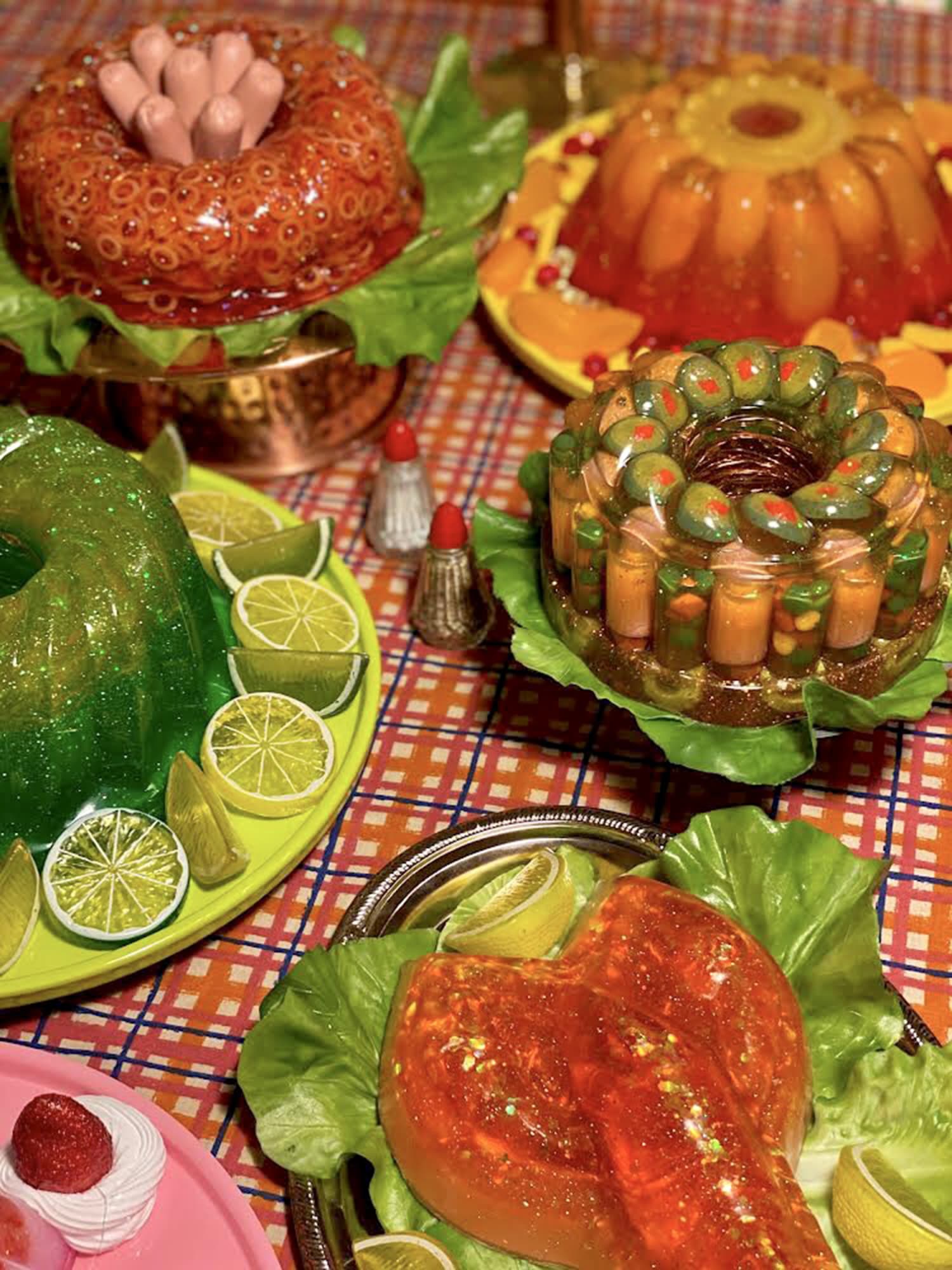The image depicts a vibrant assortment of jello desserts, arranged on a checkered tablecloth reminiscent of a 1950s dinner party. Central to the arrangement is a gradient green lime jello, presented on a green plate and surrounded by both circular and wedge slices of lime. Behind it, a conspicuous dish resembles spaghetti with Vienna sausages, intricately set on butter lettuce and a gold structure. To its right, a peach-colored jello filled with peaches sits on a yellow plate, adorned with small berries. In front of this is another jello dish, transparent and challenging to define, filled with Vienna sausages and possibly jalapenos, with red and green hues punctuating the gelatin. An orange jello with limes on lettuce, an olives-studded jello, and a faux chicken jello adorned with glitter add to the eclectic spread. Additionally, there are salt and pepper shakers centrally placed, and in the far corner, a strawberry nestled in whipped cream, completing this visually intriguing collection.